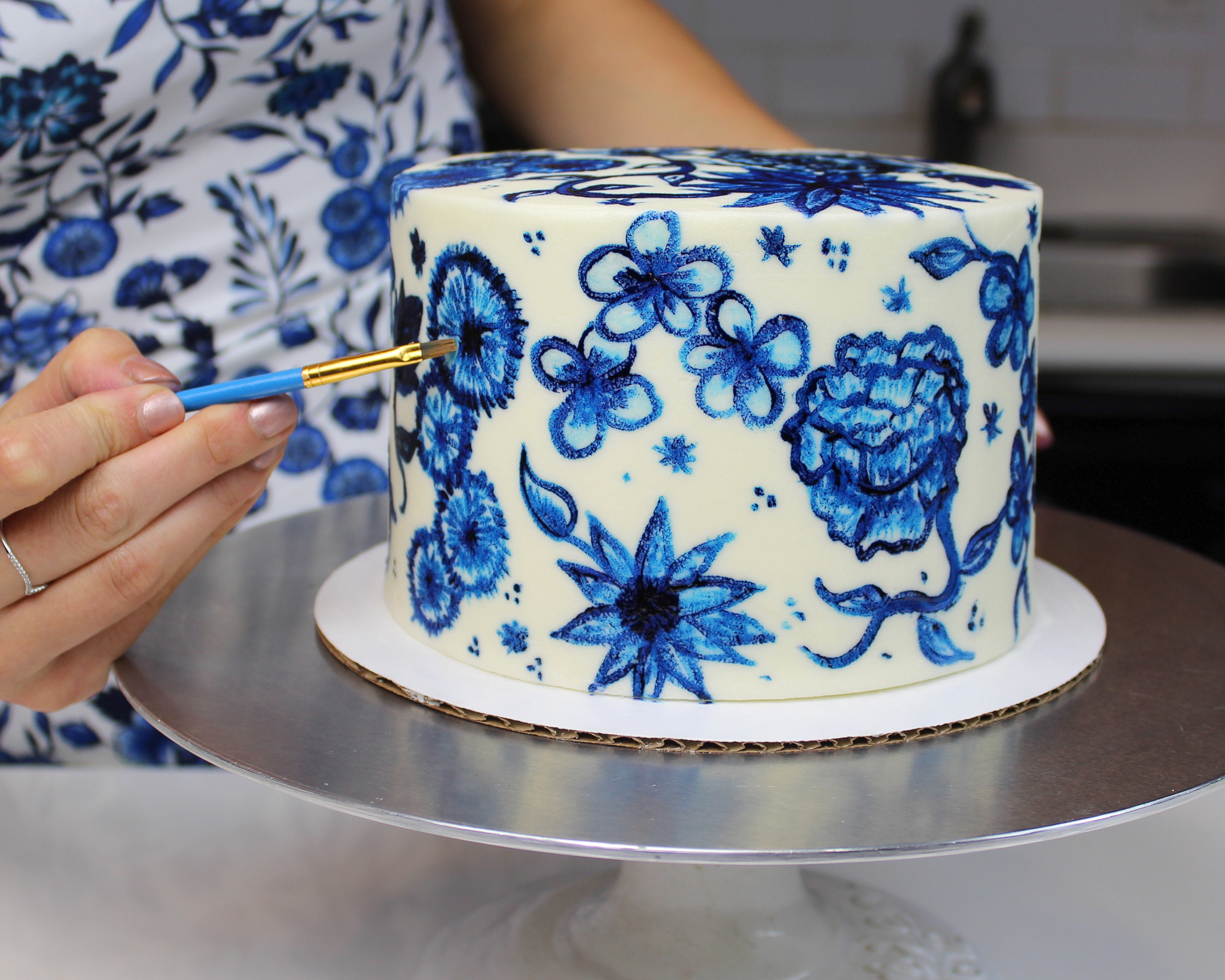This detailed close-up photograph captures a baker meticulously decorating a white, fondant-covered cake with an intricate blue floral pattern. The cake is positioned on a round, white cardboard base atop a polished, silver cake stand that rests on a gray or white table surface. The floral pattern, consisting of blue leaves, petals, and a variety of blue flowers such as daisies, carnations, and dandelion-like blooms, mirrors the baker's attire—a white dress with a matching blue floral design. The baker, of light complexion, is seen with just her left hand in the frame, holding a paintbrush with a blue handle and brass tip, delicately applying a blue petal to the cake. Her right hand, adorned with a silver filigree ring on her ring finger, is partially visible. In the blurred background, there are hints of a brick wall, a bottle, and a silver pan on nearby tables, adding to the atmosphere of a busy baking studio.